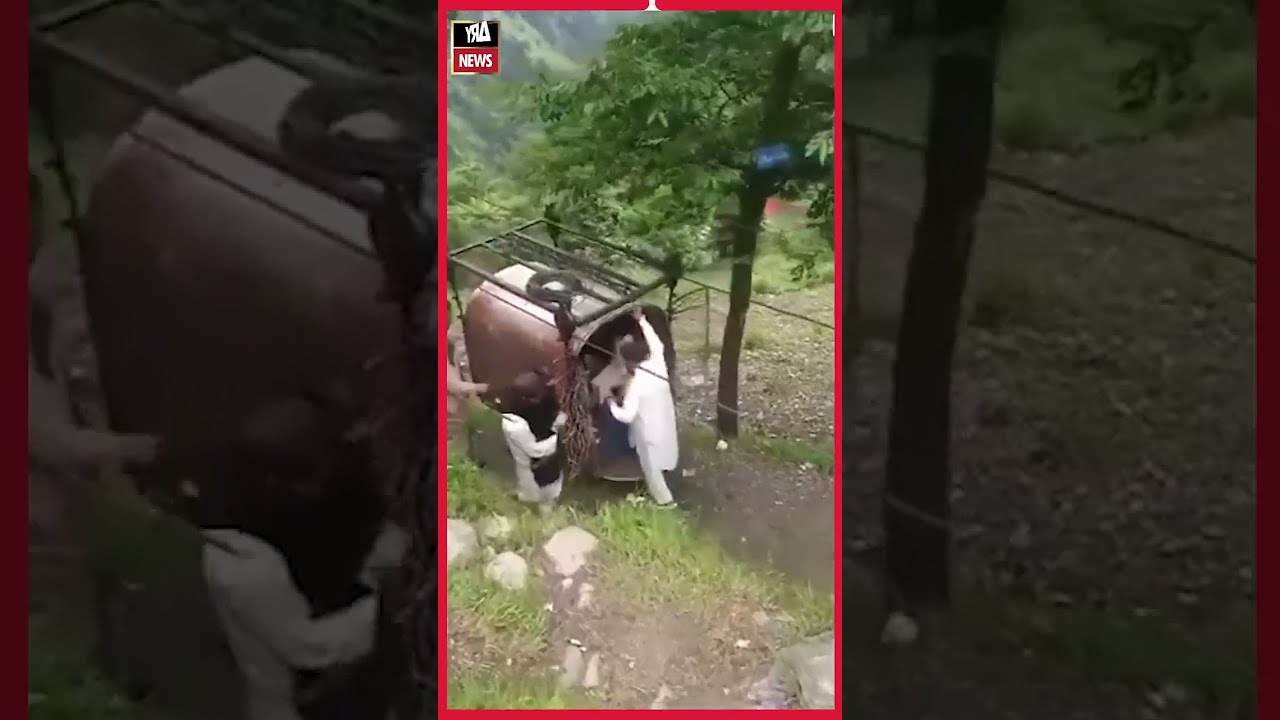In a natural setting dominated by a tall, thin-trunked tree with thick green leaves, two men dressed in white are interacting with a rust-colored container, potentially reminiscent of a cable car. The man on the right stands upright with his hand gripping the top edge of the open container, while the other man on the left is situated visibly lower. The container is encased in a black metal cage with coiled wire atop it. Lush green grass flanks both sides of a dark brown dirt walkway, which contrasts sharply with the white-colored rocks below it. The image, framed by a white border, appears to be a screenshot from a news segment, indicated by an emblem in the upper left corner comprising a black and red square, the latter marked with the word "news" in white letters. The outer sections provide close-ups: the right side focuses on the tree, and the left zooms in on the container.